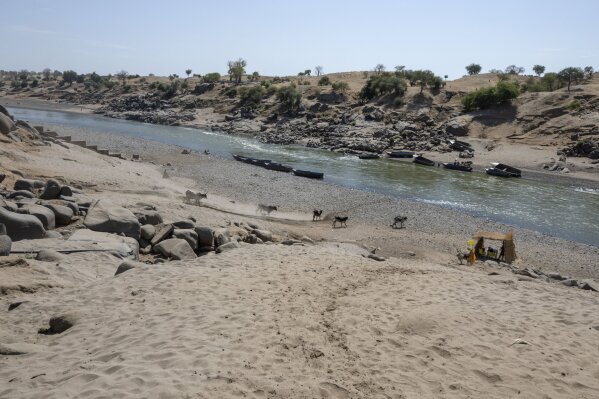In this color photograph, a meandering river with grayish-brown to greenish water cuts through a sandy desert landscape. The sand, in shades of tan and brown, sprawls across the foreground, marked by footprints and interspersed with gray rocks and scrubby vegetation. On the right side of the image, a small hut or shelter stands with indistinct figures, likely people, nearby. To the left, a rocky, almost mountainous hill is adorned with green plants, trees, and shrubbery. Along the riverbanks, dark, blurry shapes suggest the presence of boats. Scattered around, there are various animals, perhaps cows, dogs, camels, or zebras, though they are hard to accurately identify. The distant horizon reveals a desert with a stark, whitish-blue sky. The scene hints at human and animal activity, captured in neutral tones with glimpses of green and yellow.